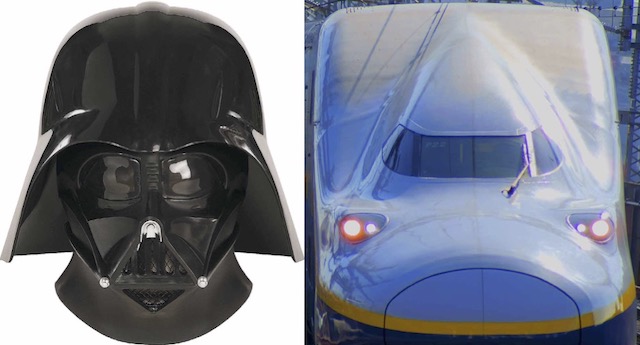This image is a composite split into two sections, divided vertically. On the left side, there is a detailed photograph of a black Darth Vader helmet from Star Wars, set against a plain white background. The helmet includes all the defining features like the iconic design that extends down to a bit of the neck, serving as a small figurine rather than wearable gear.

The right side of the image features a sophisticated vehicle, possibly an electronic train or monorail. The vehicle has a sleek, rectangular shape with a rounded nose that resembles the front of an airplane. The top of the vehicle is light sky blue, transitioning to a golden stripe in the middle, and darkens to a deeper color towards the bottom. Notable details include two prominent headlights on either side of the front, one emitting red light and the other purple, and a vivid yellow stripe along the lower part of the vehicle. The background is bare, emphasizing the subject itself.